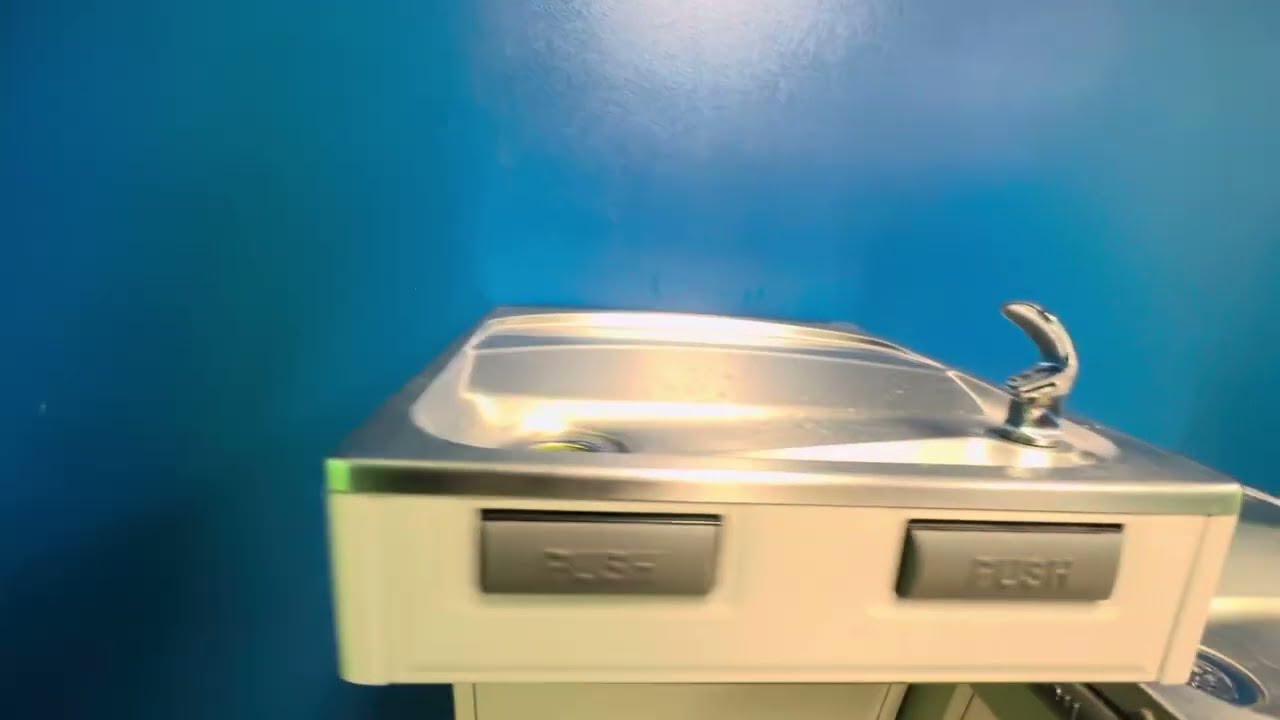The image is an indoor close-up of a drinking fountain, often called a water or bubbler depending on regional terminology. The background features a plain blue wall that is partially illuminated, possibly from the camera's flash. The fountain itself is mounted to the wall and appears to be an older model, with a light tan-colored body. Its dimensions are approximately six inches wide and three inches tall, though only the upper portion of the fountain is visible, extending from the spout to just below waist height. 

The front of the fountain has two rectangular buttons made of silver metal, both prominently embossed with the word "push." These buttons are positioned on the left and right sides of the front panel. The fountain’s basin is a shiny gray or silver metal with a slightly recessed drain visible in the left-hand portion. 

To the right of the main fountain is another shorter fixture, likely another drinking fountain, made from the same stainless steel material. Only its top portion is visible, and it features a similar basin and drain as the main fountain. The entire setup hints at an environment such as an office or a similar indoor space.